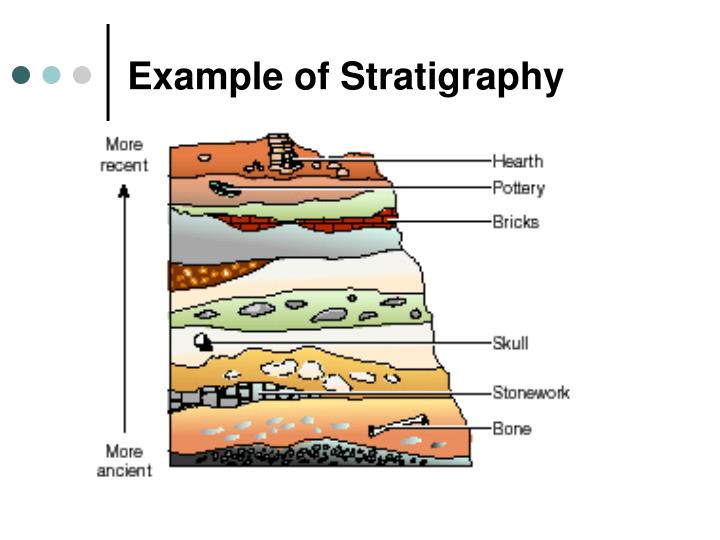This image presents a detailed cross-section diagram illustrating stratigraphy, indicating the study of layered materials in the ground. The title at the top of the image reads "Example of Stratigraphy." To the left, an arrow points upwards with labels "more recent" at the top and "more ancient" at the bottom, guiding the viewer through the chronological layers from recent to ancient times. Each layer is distinctly color-coded in shades such as peach, gold, cream, green, blue, red, and brown.

The topmost layer is labeled "Hearth," followed by "Pottery," "Bricks," and further down, "Skull," "Stonework," and "Bone." These labels denote various artifacts found within specific layers, giving a visual representation of different historical periods and the objects associated with them. The diagram effectively highlights how artifacts like pottery and bricks become progressively older as you move deeper, with items like bones and stonework indicating even older periods. The meticulous use of color and labeling provides a clear and educational illustration of stratigraphic layers and the buried treasures they hold.